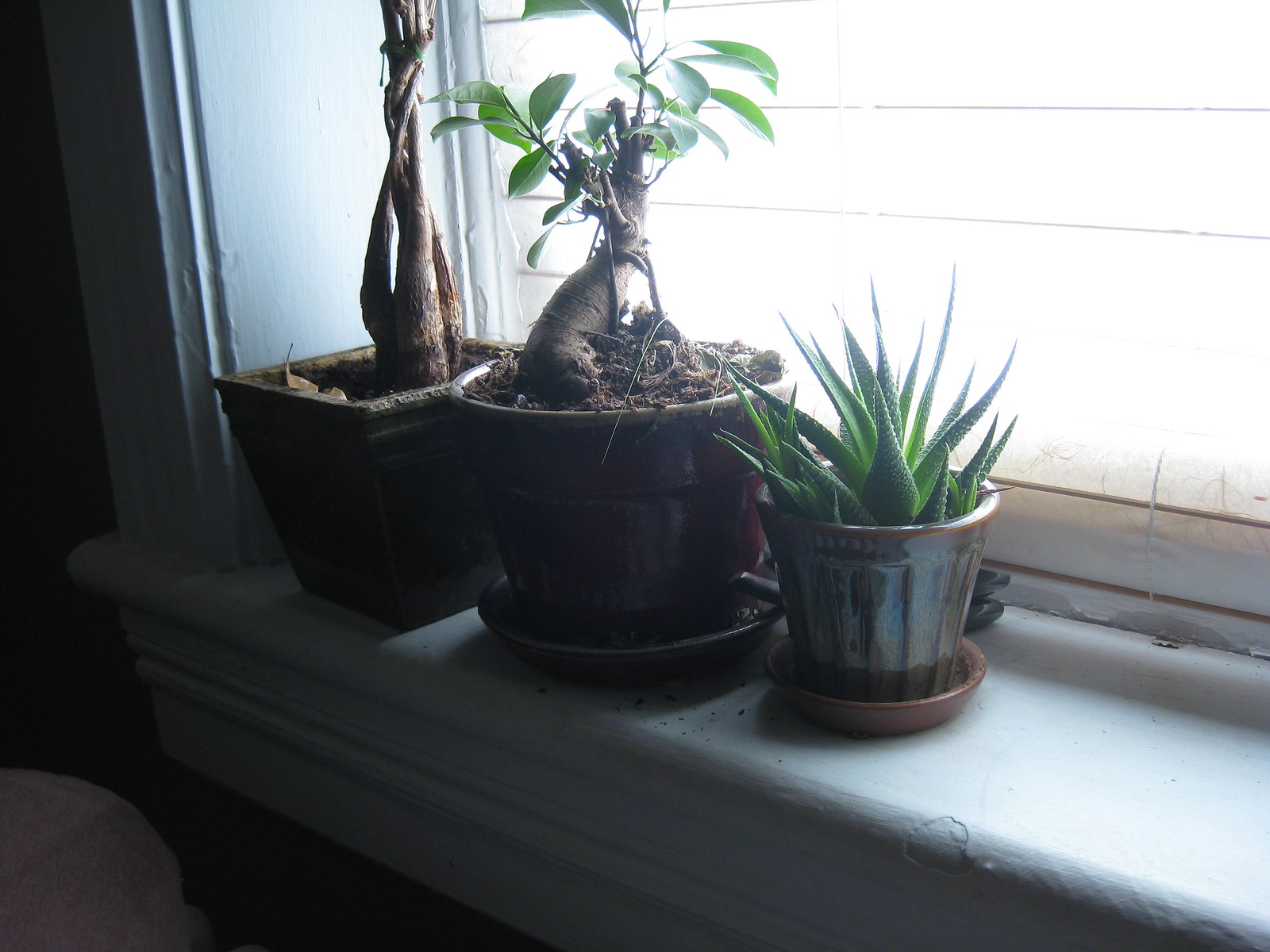This detailed photo captures a wide, white-painted windowsill adorned with three distinct plant containers. The windowsill, framed by chipped white paint, features vintage wooden blinds or a roll-down fabric covering. On the left side, there's a spacious square brown planter containing a tall stem with visible roots and no leaves. Next to it sits a round brown pot with a matching saucer, housing a plant with a prominent brown stem and green oval-shaped leaves. The smallest container is a round pot with a bronze and tan hue, also resting on a matching saucer. It contains a green, spiky aloe vera plant. In the bottom left corner of the image, there appears to be a white blanket or cloth. The overall scene presents a blend of earthy tones against the dark wall, highlighting the plants and the slightly worn but homey decor.